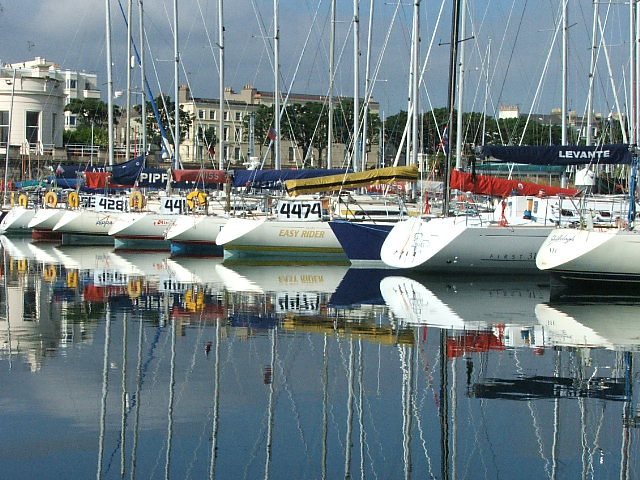This photograph captures a bustling marina filled with rows of large, white sailboats, all neatly aligned and diagonally situated. Each boat has a tall mast protruding into the cloudy, grayish sky, with some displaying covers on their sails including one that says "LEVANT." The boats strike a similar visual silhouette, though they feature unique names and colorful accents such as the prominently visible "Easy Rider." Various banners with numbers (4281, 4474) hang over the sterns, hinting at their competitive nature. The reflective water below offers a mirror-like image of the scene, adding a serene touch. In the background, residential buildings frame the marina, with a white structure on the left and a blocky, multi-windowed building on the right. Trees and a large building are visible in the far right corner, contributing to the picturesque skyline. Despite a slightly hazy atmosphere, the day appears sunny, enhancing the overall brightness and vibrancy of this detailed harbor view.